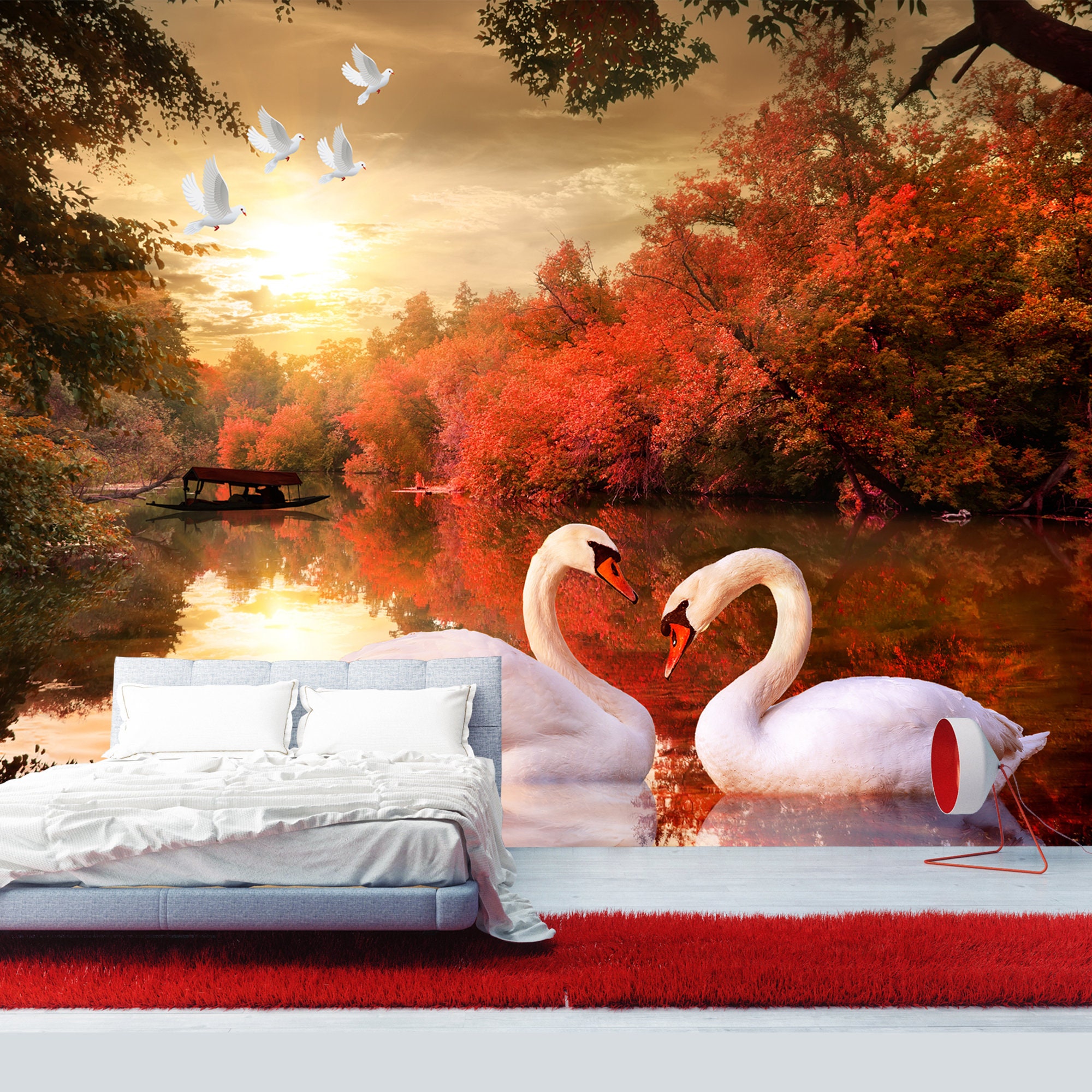The image presents an intriguing composite of a cozy bedroom scene seamlessly blended with a vibrant autumn landscape. In the foreground, a queen-sized bed dominates the lower left corner, partially but not entirely made, showing its cozy wear from use. The bed features two white pillows against a padded white headboard and a silky white blanket somewhat strewn across, revealing the sheeted mattress beneath. The bed's frame is blue, resting securely on a plush red carpet that transitions into a section of white flooring displaying a white cone-shaped space heater with a red stand and interior.

Expanding beyond this intimate bedroom setting, the scene transitions smoothly into a picturesque, classical-inspired painting of a serene pond encircled by autumnal foliage. Two elegant white swans float gracefully in the pond, their necks arched towards one another, reflecting a harmonious ambiance. The water mirrors the vivid surroundings—red and orange shrubs and trees dominate the right side, echoing their rich hues in the pond, while the left side showcases more traditionally green foliage. Above, a luminous yellow sky, lit by a bright sun partly hidden by clouds, bathes the scene in a warm glow, with four white birds soaring gracefully overhead. The serene pond also features a small, covered canoe, adding to the pastoral charm.

This composite image, with its juxtaposition of a cozy bed and an idyllic autumn landscape, creates a nuanced and inviting tableau, likely suggesting themes of comfort and tranquility, possibly intended as an advertisement for a bed or a luxurious comfort suite.